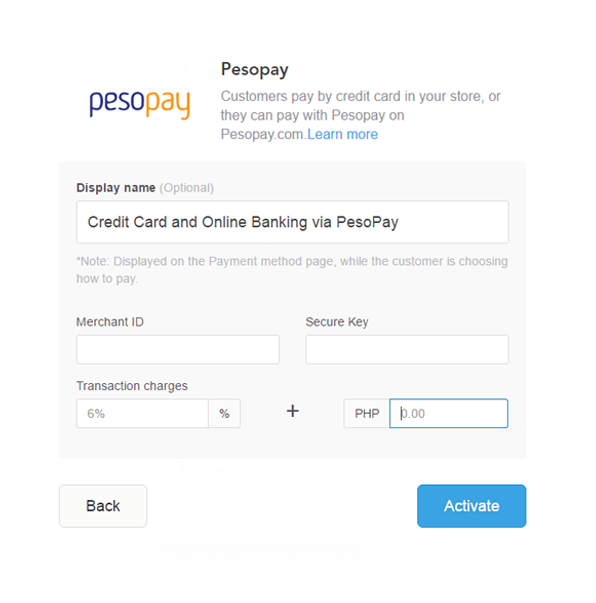This is a detailed screenshot of the PesoPay website, a platform designed for facilitating online payments. The name "PesoPay" is prominently displayed at the top center in black. On the right side, the name "PesoPay" appears again, but this time, "Peso" is in blue and "Pay" is in orange. Next to this logo, there is a brief description: "Customers can pay by credit card in your store, or they can pay with PesoPay on PesoPay.com. Learn more."

Below this description, there is a large gray box extending almost to the bottom of the screen. Inside this gray box, several sections provide information and options related to payment settings. The first section includes an optional field labeled "Display Name." Below this, a white box contains the text "Credit Card and Online Banking via PesoPay." Following this, a note clarifies that this text will be displayed on the payment method page while the customer is choosing how to pay.

Further down in the gray box, fields are provided for entering a "Merchant ID," a "Secure Key," and details about "Transaction Charges" along with the indication "plus PHP." Another box appears to summarize the total charges.

Beneath the gray box, there are two buttons: one labeled "Back" and another labeled "Activate."

This screenshot highlights PesoPay's user interface for merchants, showcasing the options for configuring payment methods and providing a glimpse into how the service operates to support e-commerce transactions.